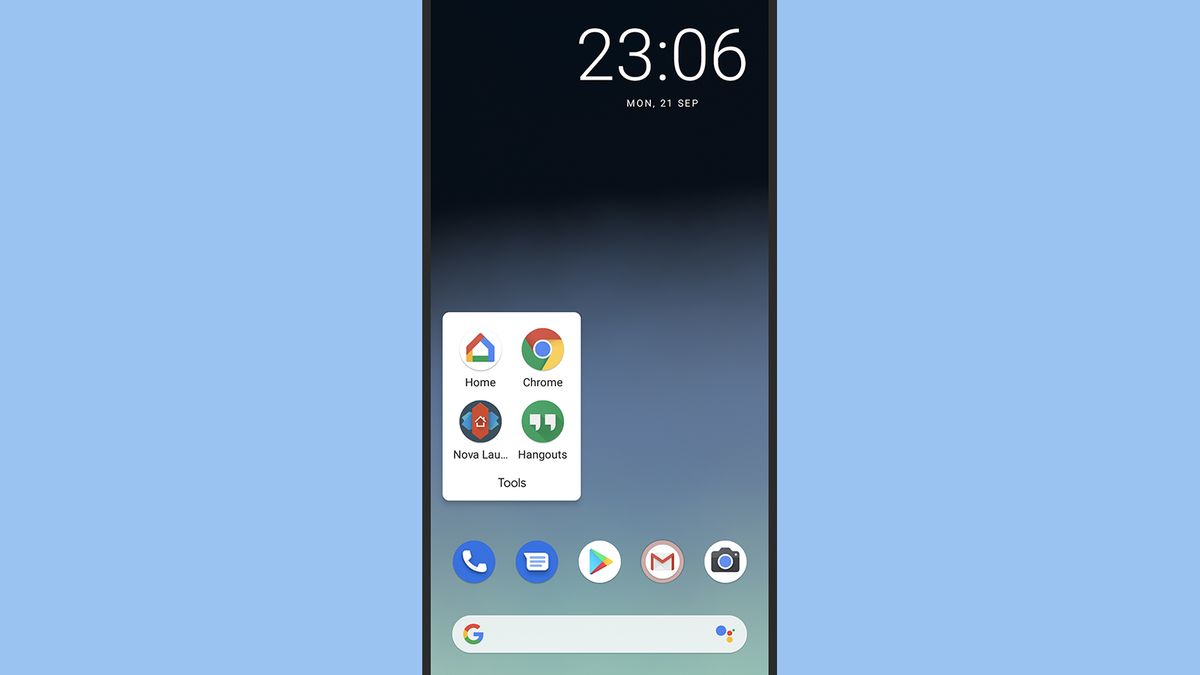This image is a screenshot from a smartphone displayed against a blue background. The phone's screen is divided into three distinct color sections: the top is black, the middle is blue, and the bottom is blue-green. In the top right corner, the time is prominently displayed in large white numbers as "23:06" (11:06 PM), with the date "Mon, 21 Sep" in smaller white letters directly beneath it.

In the central part of the screen, there is a white area featuring various navigation icons for accessing different apps on the phone. These icons include "Home" for the main screen, "Chrome" for the web browser, and several other icons that are not clearly distinguishable.

At the bottom of the screen are additional icons for essential functions such as making phone calls, texting, accessing email, and taking photographs.